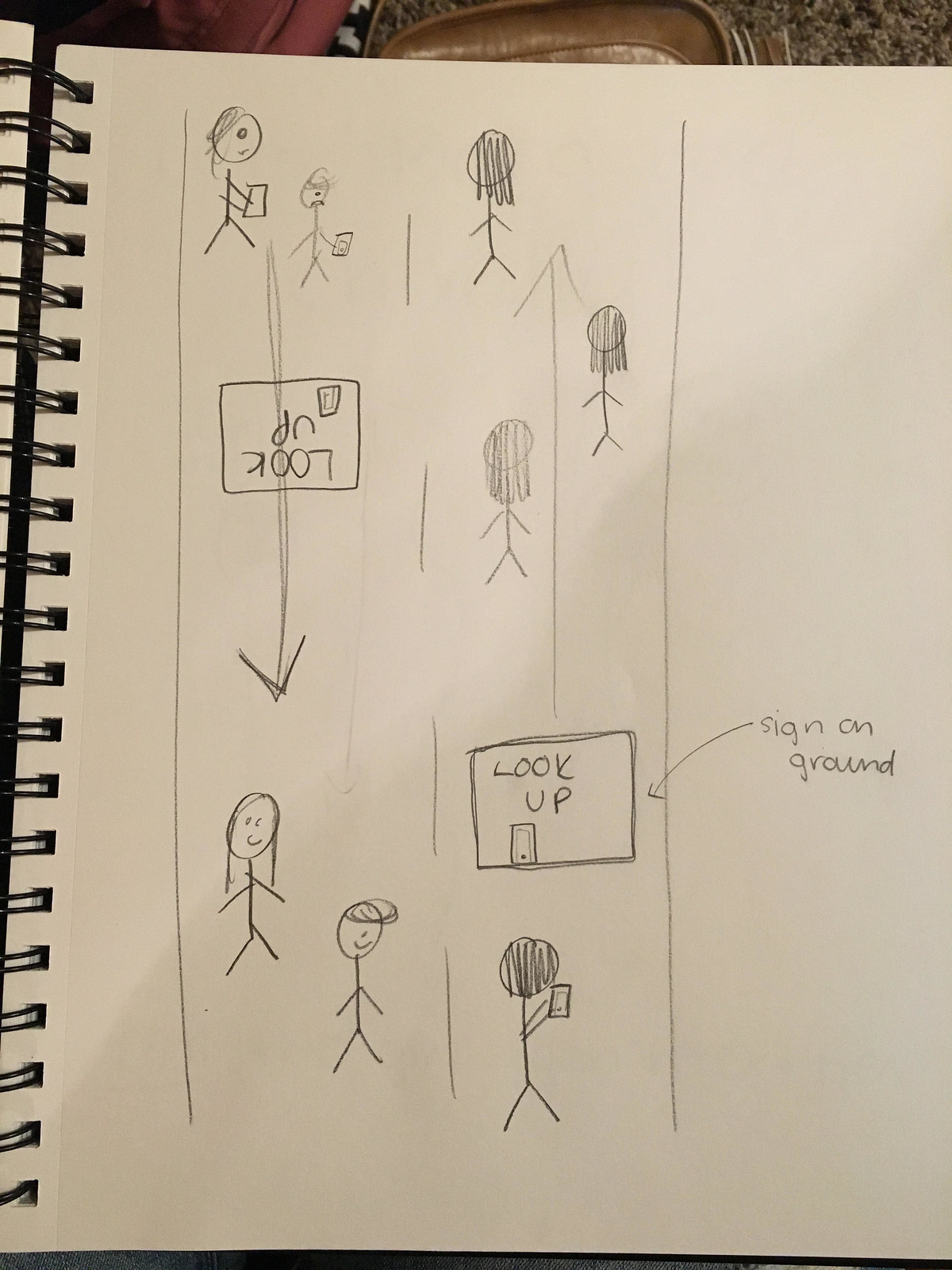The image is a photograph of a line drawing on a white, spiral-bound notebook, with artificial lighting giving the paper a beige tint. The right page of the notebook contains a detailed sketch primarily created in black pencil. The drawing features numerous stick figures in various arrangements. At the bottom, several stick figures are walking towards the right, accompanied by a box labeled "look up" with a small door underneath it. An arrow points to this box from the far right, with a "sign on ground" notation next to it. 

Above this section, more stick figures are depicted. Three at the top have long hair and simple stick bodies, and they appear to be looking away from the viewer. One figure is holding a rectangle and stands next to a smaller figure. An envelope-shaped arrow with the words "look up" points downward towards these figures, indicating a connection between the upper and lower groups. Additionally, on the left side of the page, an inverted "look up" sign points downwards, and near this sign, stick figures appear to be holding objects resembling smartphones.

Overall, the complex arrangement of stick figures, directional arrows, and labeled signs, combined with various visual elements, suggests a narrative or instructional theme within the drawing.